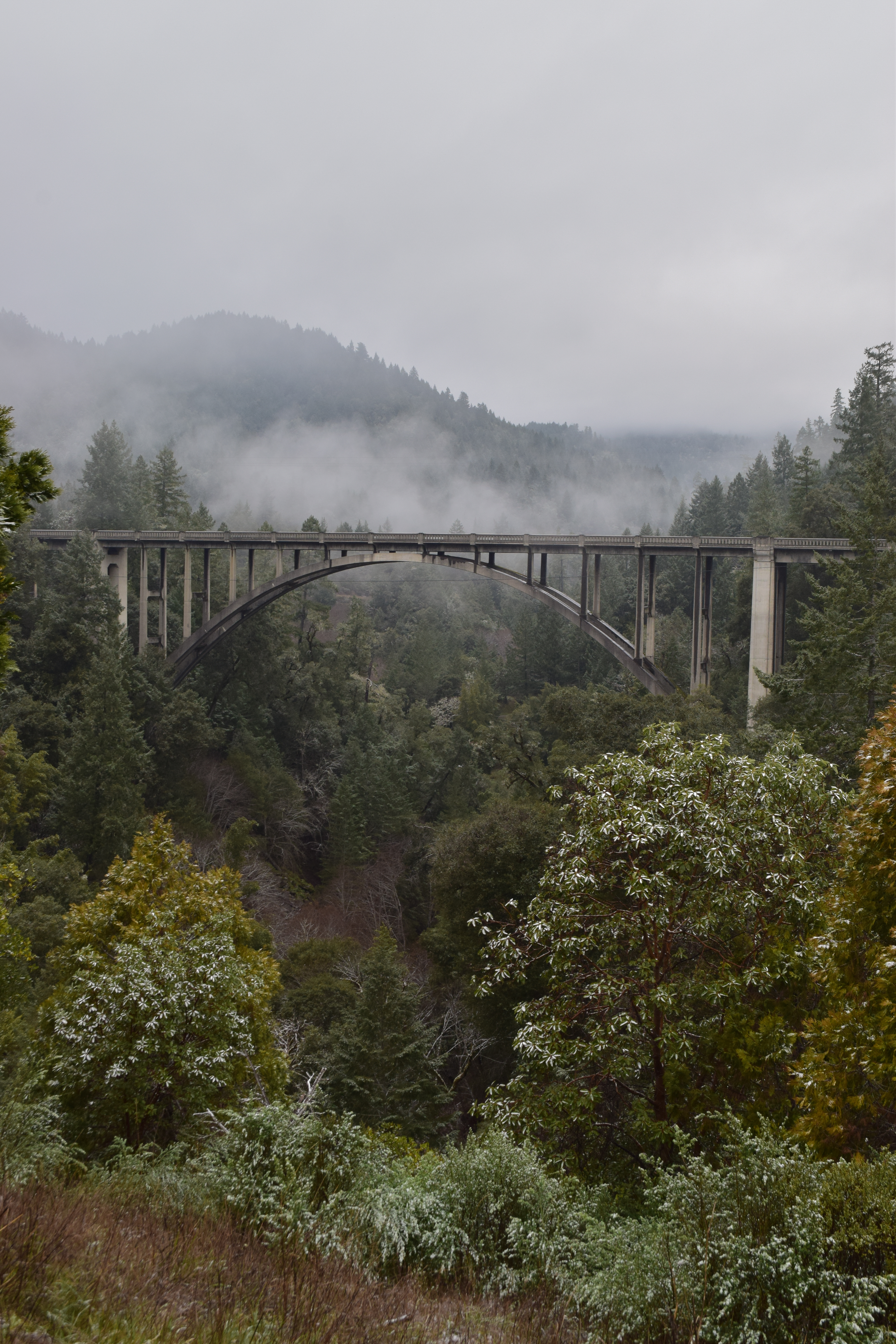A scenic bridge spans a deep gorge in West Virginia, blending harmoniously with the lush, verdant landscape. The elegant, arched structure, likely composed of reinforced concrete, stands confidently amidst a sea of green trees and plant life that covers the valley floor and climbs the distant hills and mountains. The atmosphere carries a hazy, foggy quality, enshrouding the backdrop in a gentle mist that adds a layer of mystique to the scene. Clouds hang overhead, casting a soft, diffused light that indicates an overcast day. While most of the foliage remains vividly green, a few trees hint at the upcoming change of seasons, suggesting early fall. This iconic bridge, renowned for its picturesque charm especially during the fall, when the area bursts into vibrant autumnal colors, showcases the timeless beauty of West Virginia’s natural landscape.